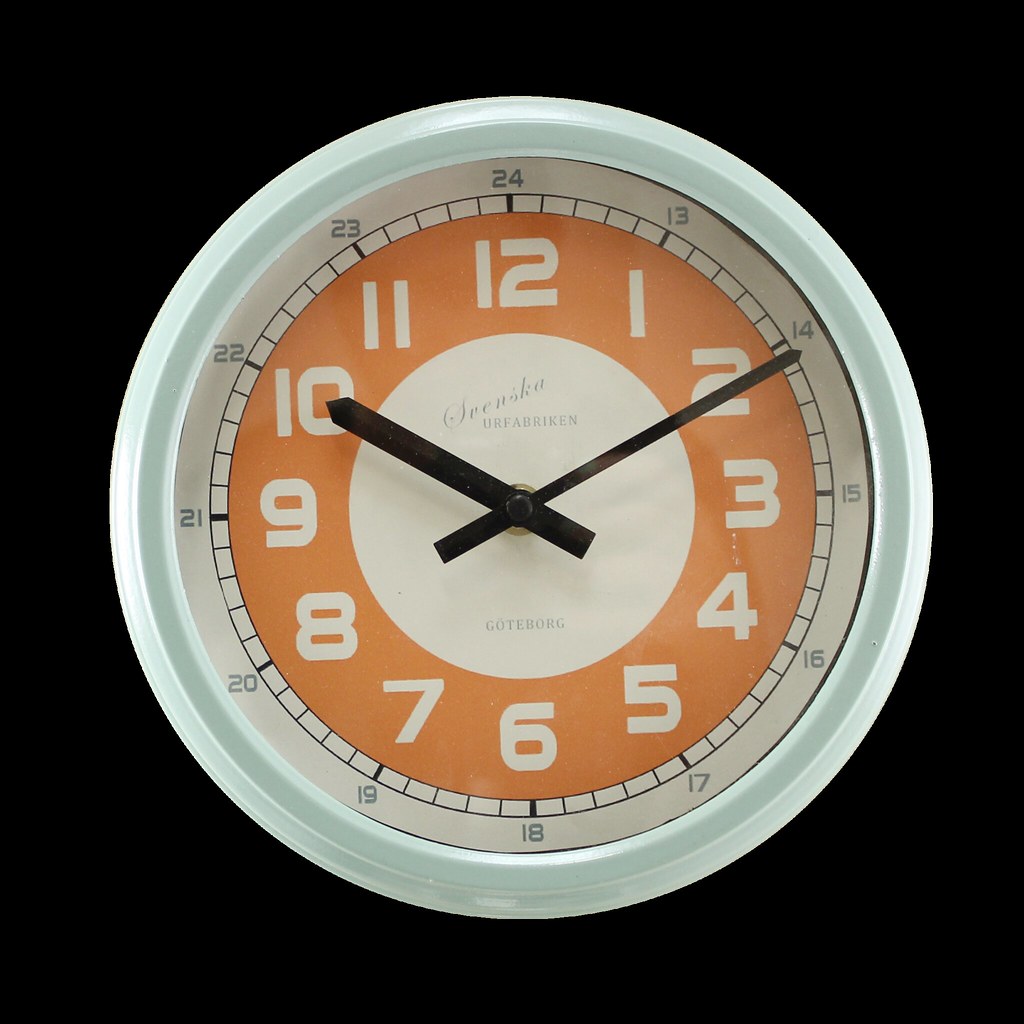This is a photograph featuring a vintage-style round clock set against a black background. The clock has a white body with a slightly reflective surface that accentuates its contours. The clock face itself has a rich orange background adorned with white numerals, providing a striking contrast. Encircling this orange area, additional gray numbers add to the detailing. The clock hands are black, standing out prominently against the white and orange segments of the face. The center of the clock bears a white section, adding to the visual interest, while gray font details overlay and appear underneath the clock hands. The design and typography evoke a 1970s aesthetic, contributing to the clock's vintage charm. The image is crisp and clear, highlighting the intricate details of this nostalgic timepiece.